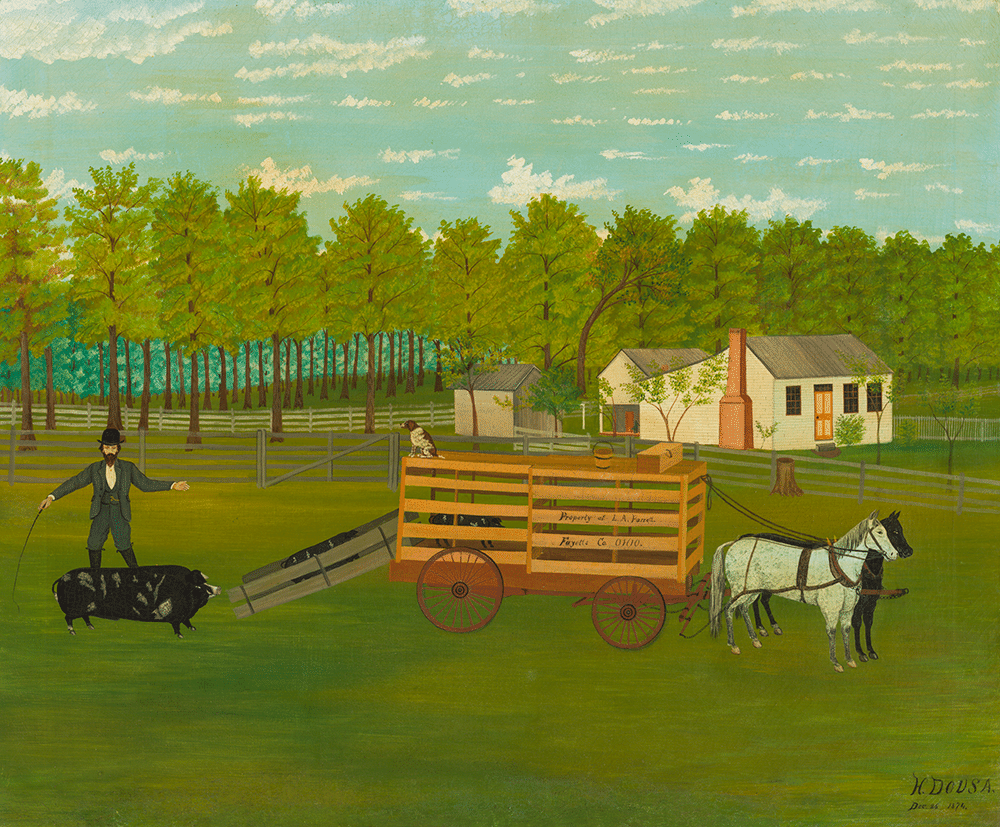The image is a detailed painting of a pastoral farmland scene. In the foreground, there is a wooden carriage with large wheels, pulled by two horses. A man, wearing a hat and holding a whip, stands behind the carriage, guiding a ramp where several pigs are being loaded into the wagon. Another pig can be seen inside the cart. A small dog sits on top of the carriage, observing the activity. The background features expansive green fields, lush trees of uniform size and color, and a white house with a chimney. A blue sky filled with white clouds completes the idyllic setting. The painting, characterized by its folksy style, is signed in the bottom right-hand corner by an artist whose name is somewhat illegible but appears to be "H-D-O-U-S-A." The cart has "Property of L.A." and "Fayette County" inscribed on it, with further details that are not fully legible. The overall composition suggests a serene, rural atmosphere.